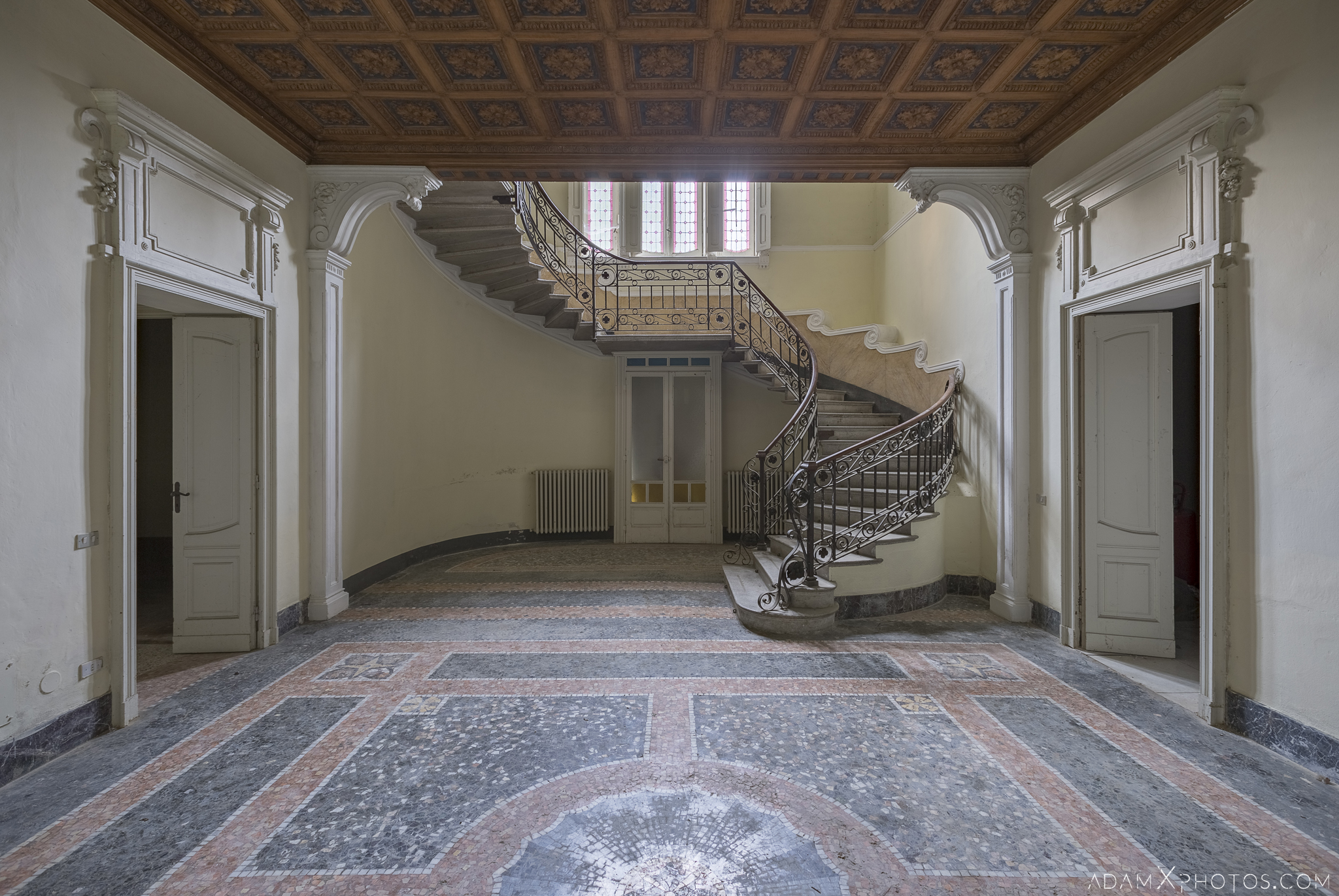The image features the grand, empty interior of a mansion or villa, highlighting an impressive, sweeping curved staircase with a fancy black metal railing that ascends to the second story. The striking staircase is positioned towards the back of the room, where it curls gracefully around a large window at the top. The spacious room boasts an ornately inlaid floor that resembles a large Persian rug, possibly made of marble or mosaic. 

On either side of this grand foyer are wide double doors with intricately carved, ornate woodwork frames, reminiscent of an elaborate fireplace surround, complete with decorative transom panels above. The ceiling, adding to the grandeur of the room, is elaborately coffered with light wood rectangular designs or perhaps intricately carved mahogany or teak.

Behind the staircase are two tall windows integrated into a door, leading to an area which might feature a dumbwaiter flanked by radiators, suggesting practicality amidst elegance. The left doorway is open with a white door, while the right doorway also features a white door, elegantly tying the space together. The absence of furniture leaves the room feeling possibly abandoned or in the process of being moved into, emphasizing its architectural splendor and intricate details.